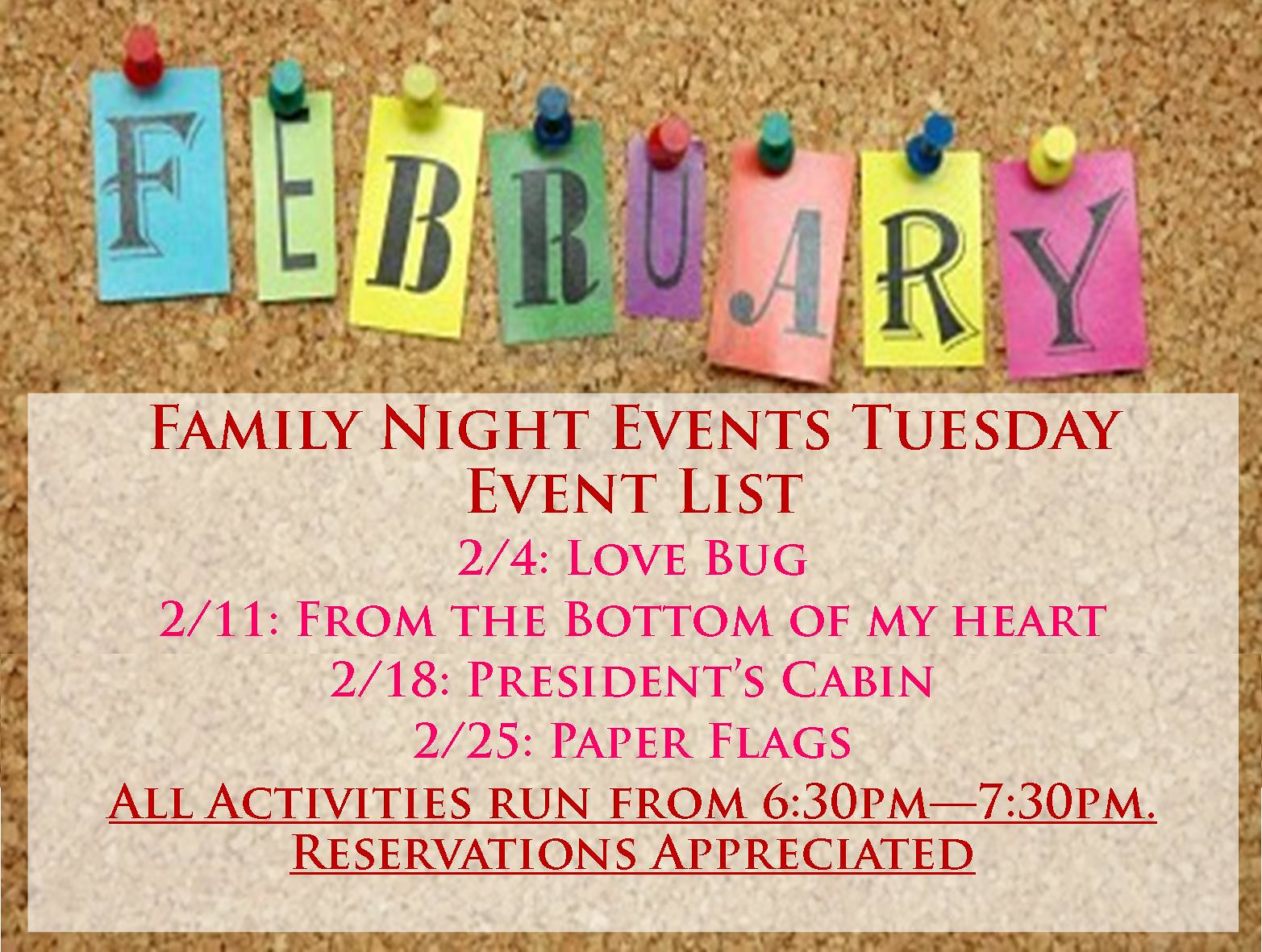This color image showcases a close-up of a bulletin board made of brown cork. Across the top of the board, the month "February" is spelled out with individual letters cut from different colored paper and pinned with various colored pushpins—blue, green, yellow, and purple. Each letter (F-E-B-R-U-A-R-Y) is uniquely colored: the F is on a blue background, the E on green, the B on yellow, the R on green, the U on purple, the A on pink, the second R on yellow, and the Y on purple. Below this, on what appears to be a Times New Roman font banner, it reads: "Family Night Events, Tuesday Event List." It lists the following dates and events: February 4th - Love Bug, February 11th - From the Bottom of My Heart, February 18th - President's Cabin, and February 25th - Paper Flags. The notice further specifies that all activities run from 6:30 PM to 7:30 PM, and reservations are appreciated.